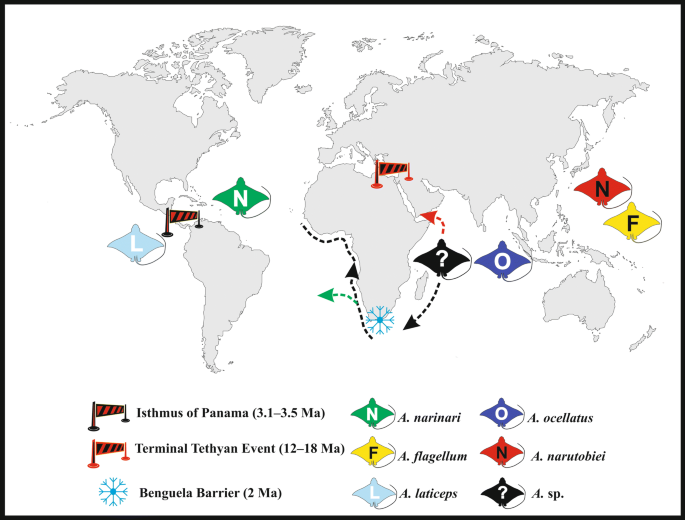This image illustrates an intricate artist's map of the world's continents, featuring a white background bordered in black and laid out in landscape mode. It includes a variety of vividly colored emblems and arrows indicating waterways and migration routes. The map prominently depicts stingray-shaped icons in light blue, green, yellow, red, black, and blue, signifying different regions and routes. 

Key locations identified are the Isthmus of Panama, marked with red and black striped goal posts, highlighting the geological event from 3.1 to 3.5 million years ago. The Terminal Tethyan Event, occurring between 12 to 18 million years ago, is marked with orange and blue goal posts at the top of Africa. The Benguela Barrier, marked with a bright green snowflake circle, situated near the Cape of South Africa, represents an event from 2 million years ago.

Additional elements include dotted lines with arrows outlining the base of Africa, and various site-specific identifiers such as Nareneri, Plagellum, Latticeps, Ocellatus, Nehru, Tobai, and SP. Symbols like NFO, question marks, and flags are distributed across the map, with constellation-like formations resembling stingrays.

Overall, this complex map not only charts geographic features but also integrates a legend at the bottom to decode the colorful stingray emblems, symbols, and pathways, depicting a comprehensive visual narrative of historical canal locations, movements, and significant geological events.